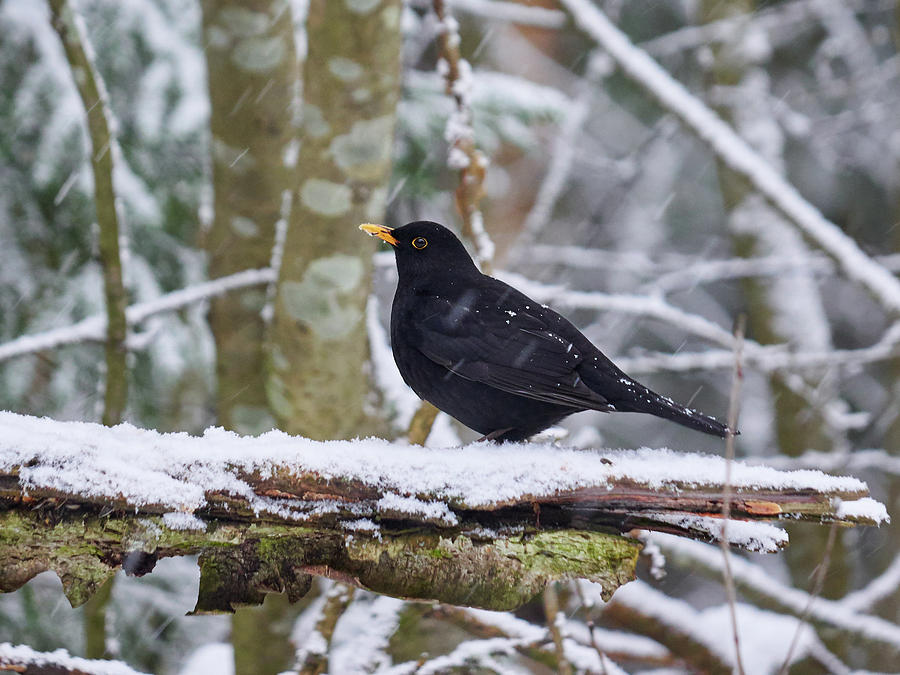The image captures a serene winter scene in a wooded area, focusing on a small black bird with a striking yellow beak and yellow eyes outlined with black pupils. The bird, perched on a frosted tree branch, gazes contemplatively to the left. Snow gently falls, visible as streaks in the image, giving a sense of motion. In the background, the entire setting is blurred, emphasizing the bird while revealing an intricate network of tree branches and a thick tree trunk, all blanketed in a light layer of snow. The quiet beauty of this moment reflects the bird's solitary presence amidst the frosty landscape.